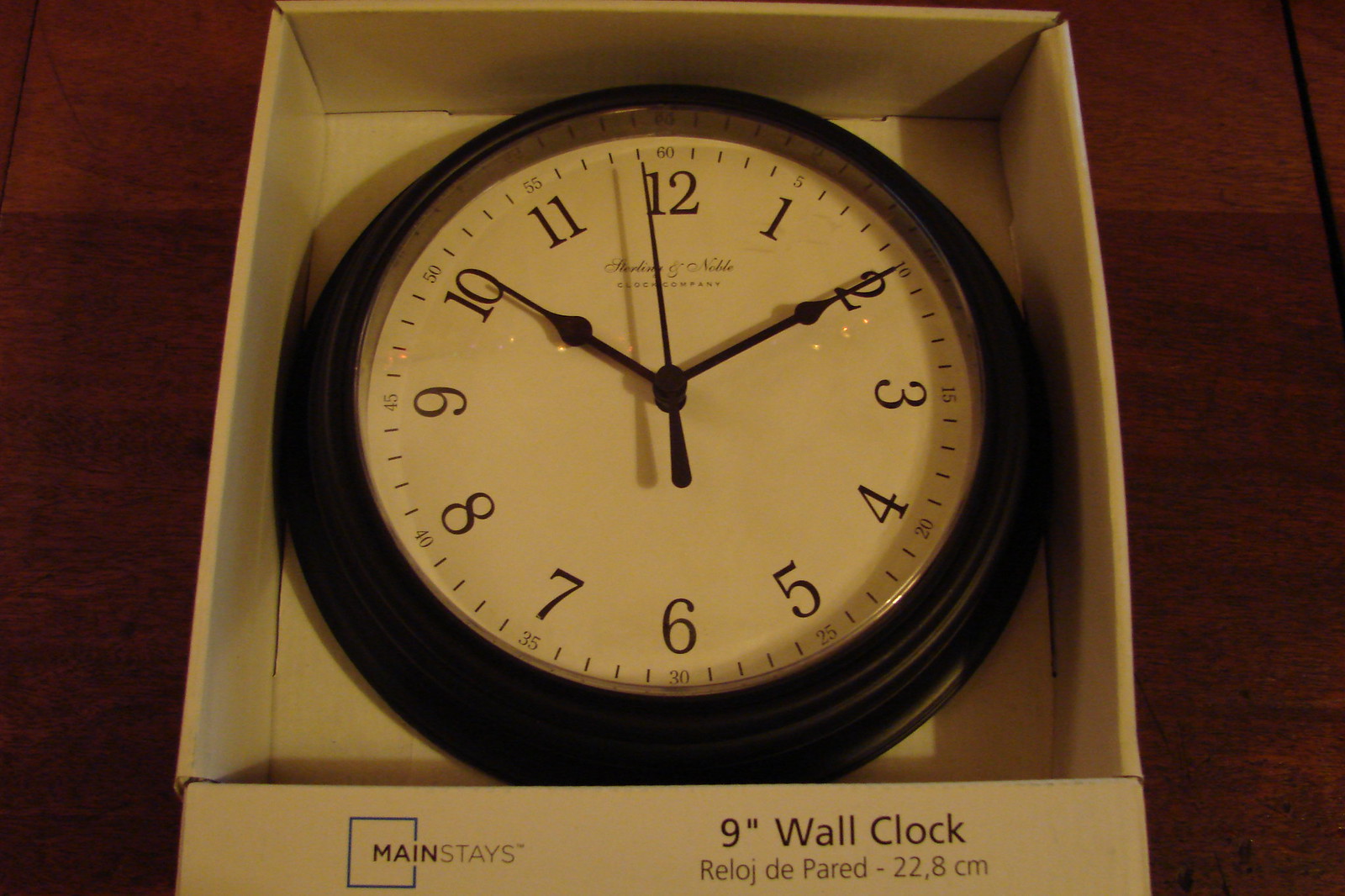This photograph depicts a circular wall clock still inside its store packaging. The clock features a black frame, which seems to be made of either plastic, wood, or metal, with a white clock face. It displays black numerals for each hour, black minute and second markers, and black hour, minute, and second hands. The hands are set to 10:10 and 59 seconds. Surrounding the clock are clear minute demarcations with small dashes between the numbered hours. 

The clock is housed in a white square box, which is positioned on a dark brown wooden table. The packaging prominently displays the brand "Mainstays" on the bottom left, with "Maine" written in bold black text inside a blue square, followed by "stays" in black text. The packaging also indicates the size of the clock as "9 inch wall clock," and provides a metric measurement of "22.8 centimeters," along with the Spanish translation, "relo de pared."